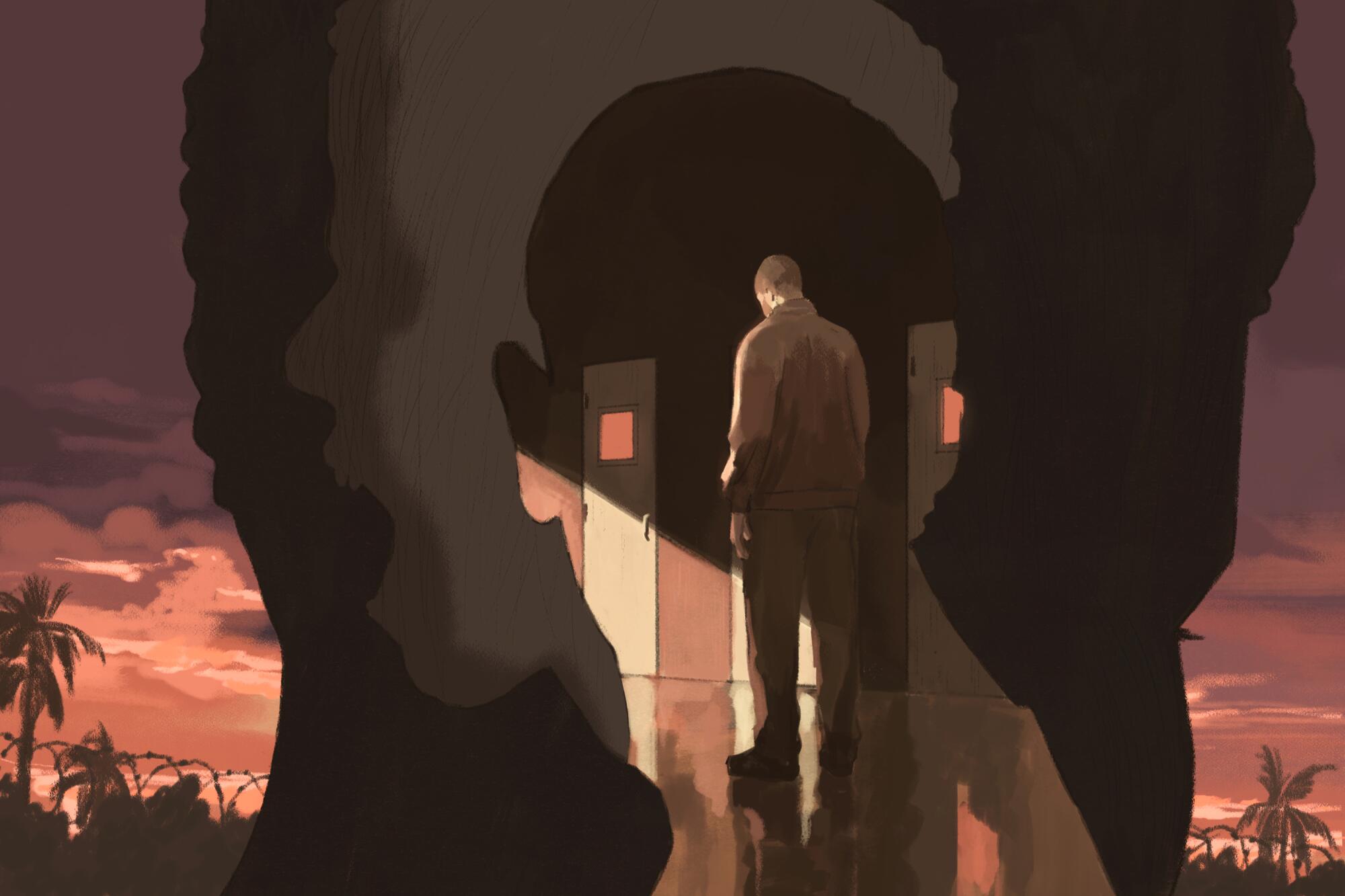The image is a minimalist composition rendered in dark brown, rust brown, and light tan tones. Dominating the canvas is a dark outline silhouette of a man's head, which takes up the majority of the space. Inside this silhouette, the central focus shifts to reveal another shape of a head. To the left side of this inner head, an ear is visible, and within it, a man stands on a shiny brown and tan floor. The man, dressed in a tan jacket and tan pants, faces away from the viewer with his head bent down as if in deep thought. His short-cropped hair and brown loafers are discernible. To his right, three tan doors each have a small square window emitting an amber or red light. The background sky transitions from rusty brown to tangerine and cream shades, adding dramatic contrast to the silhouetted palm trees lining the base of the image. Within this layered artwork, additional elements appear: a third silhouette of a younger person, mouth open as if screaming or singing, and two prominent windows just below eye level suggest both depth and narrative complexity. The scene exudes a watercolor, cartoony style, evocative of a video game still shot, with earthy, dark to light red tones throughout.